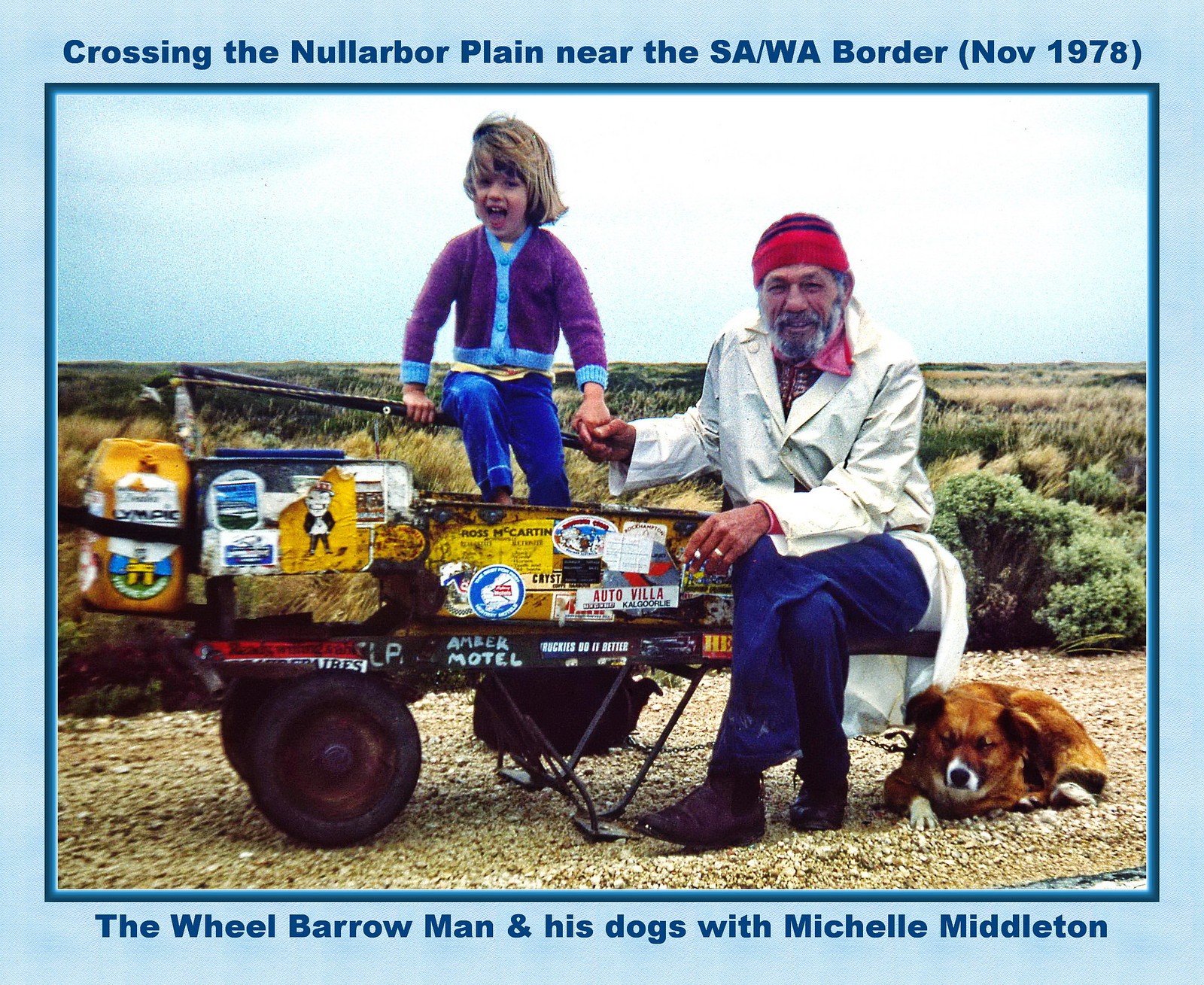This photograph, roughly 40-45 years old and framed in light blue with text labels at the top and bottom, captures a heartwarming scene from November 1978 on an overcast day. The top label reads "Crossing the Nullarbor Plain near the SA-WA border (Nov 1978)" and the bottom label says "The Wheelbarrow Man and his dogs with Michelle Middleton." The image shows an older man, known as the Wheelbarrow Man, seated on a stool next to a wheelbarrow. He wears a red beanie with blue at the top, a cream-colored jacket, a red and pink patterned shirt, blue pants, and brown leather shoes. His right hand holds the left hand of a smiling little girl, identified as Michelle Middleton, who is climbing onto the wheelbarrow. Michelle has chin-length blonde hair, a purple sweater with blue trim, and blue pants. The wheelbarrow is rusted and covered in stickers, with "Amber Motel" written on its side, and contains bundles of hay and pallets of a drink. A red-colored dog with a chain, eyes closed and seated next to the man, completes the scene. They are situated on a mulch surface with a grassy prairie that stretches into the horizon, forming a picturesque backdrop.